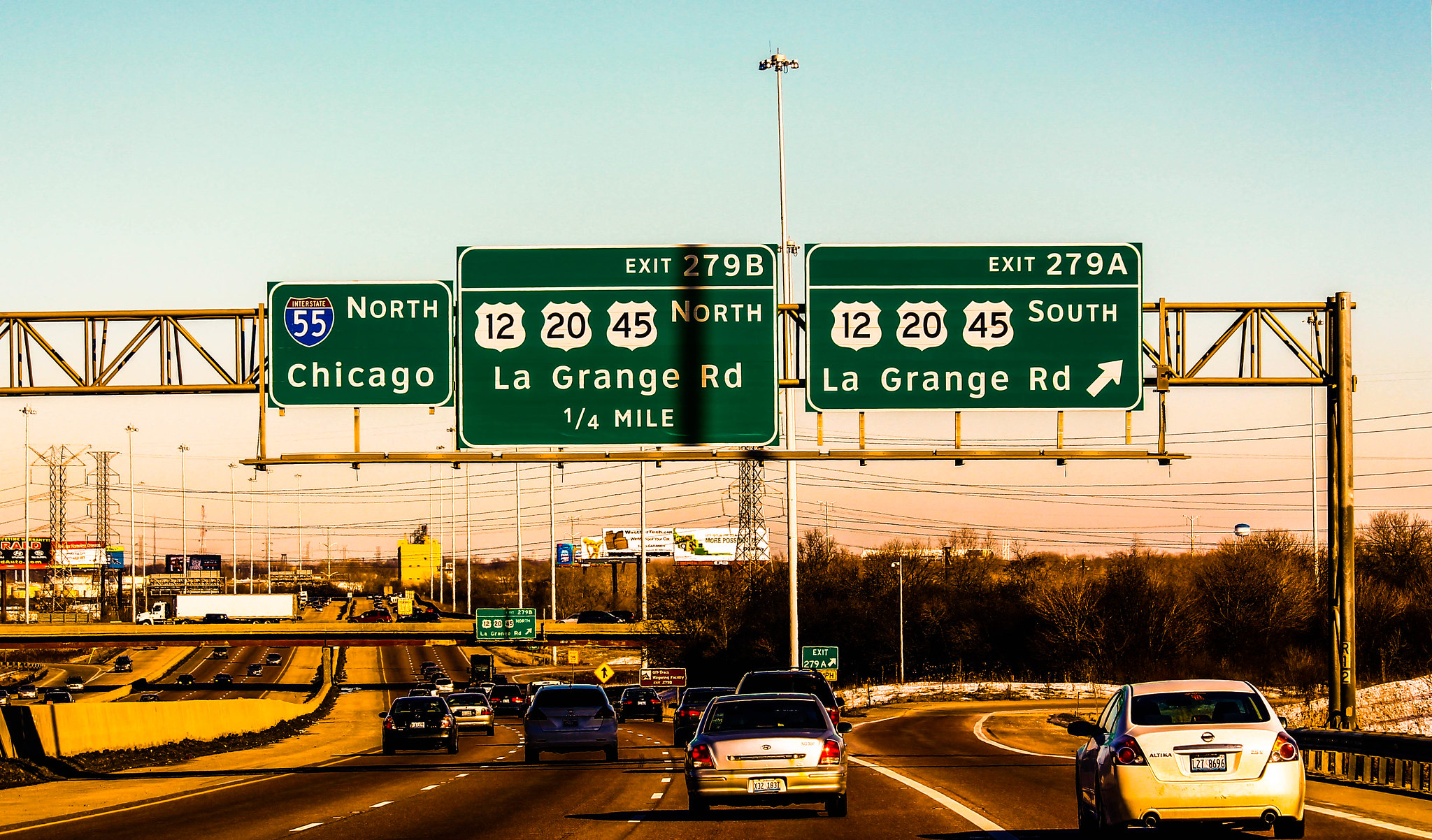The image depicts a busy interstate highway under a mostly clear blue sky with a hint of white near the horizon. Spanning across the highway is a prominent metal golden frame, adorned with three green directional signs. The leftmost sign directs travelers to Interstate 55 North towards Chicago. The middle sign marks Exit 279B and lists upcoming routes for Interstates 12, 20, and 45 North to LaGrange Road, just a quarter mile ahead. The third sign, on the right, indicates Exit 279A for Interstates 12, 20, and 45 South, also leading to LaGrange Road, with an arrow pointing to the right. Below, several cars, including a light-colored vehicle on an exit ramp, traverse the multiple lanes of the roadway. In the background, an overpass accommodates a white semi-truck and the distant silhouette of a building, possibly reflecting sunlight. The scene includes green and yellow hues interspersed with the dominant blue and white of the sky, capturing a typical bustling highway atmosphere.